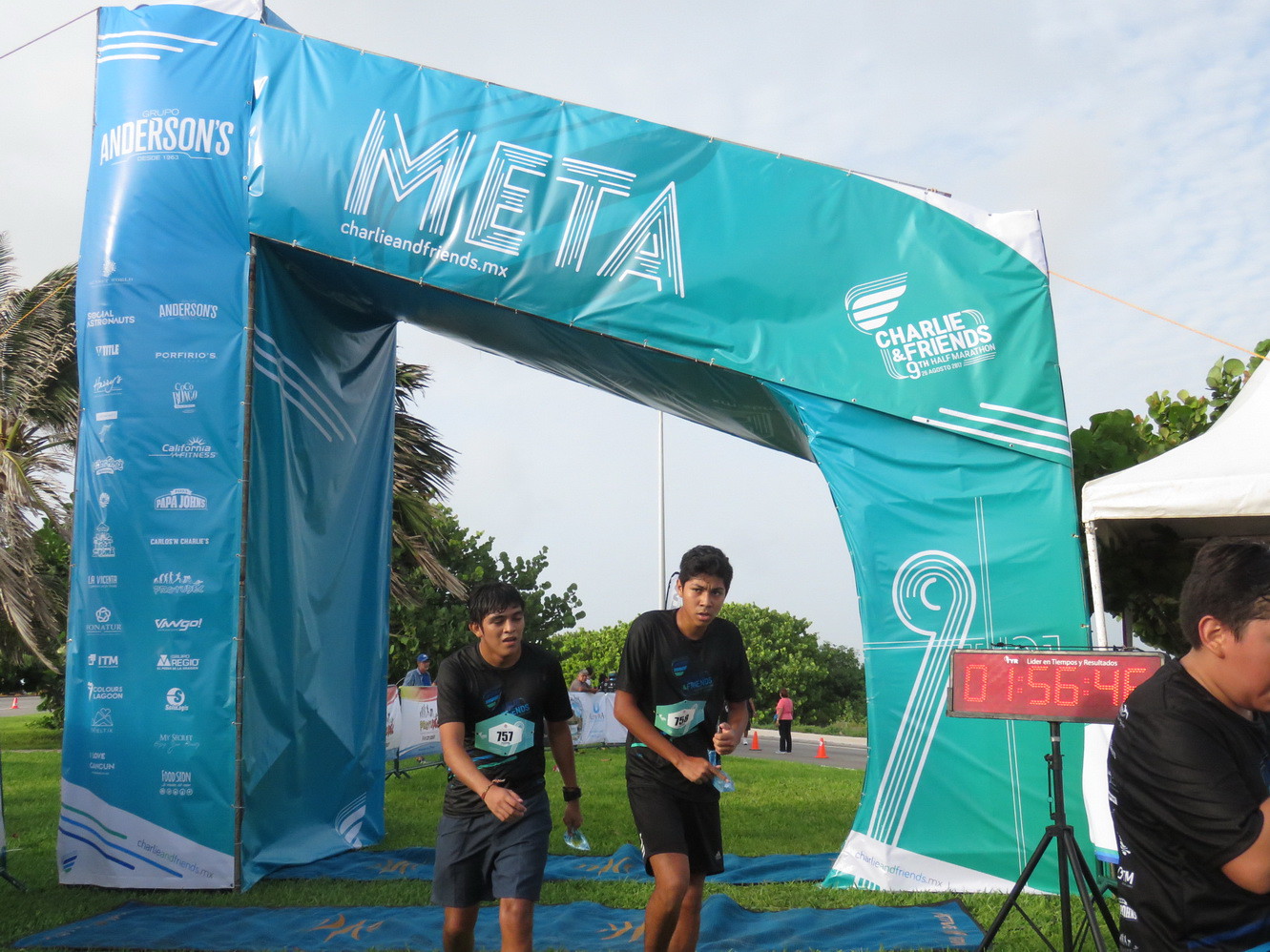In the picture, two boys, drenched in sweat, are crossing the finish line of a race. Both boys are wearing black shirts and dark shorts, with visible race numbers on their chests—one clearly reads 757, while the other number starts with a 7 but is partially obscured. The finish line itself is an arced, colorful structure that transitions from blue to green and prominently displays the text "META Charlie and Friends dot MX" along with logos of multiple sponsors such as Papa John's and Anderson's. A digital clock to the right shows a time of 1 hour, 56 minutes, and 46 seconds. In the background, you can see a grassy field, some trees, and scattered clouds in the sky. The finish line area also has blue tarps laid on the ground. There is a man partially cut off by the photo, standing near the timer with his arms at his sides, and the overall scene is set outdoors in the middle of the day.